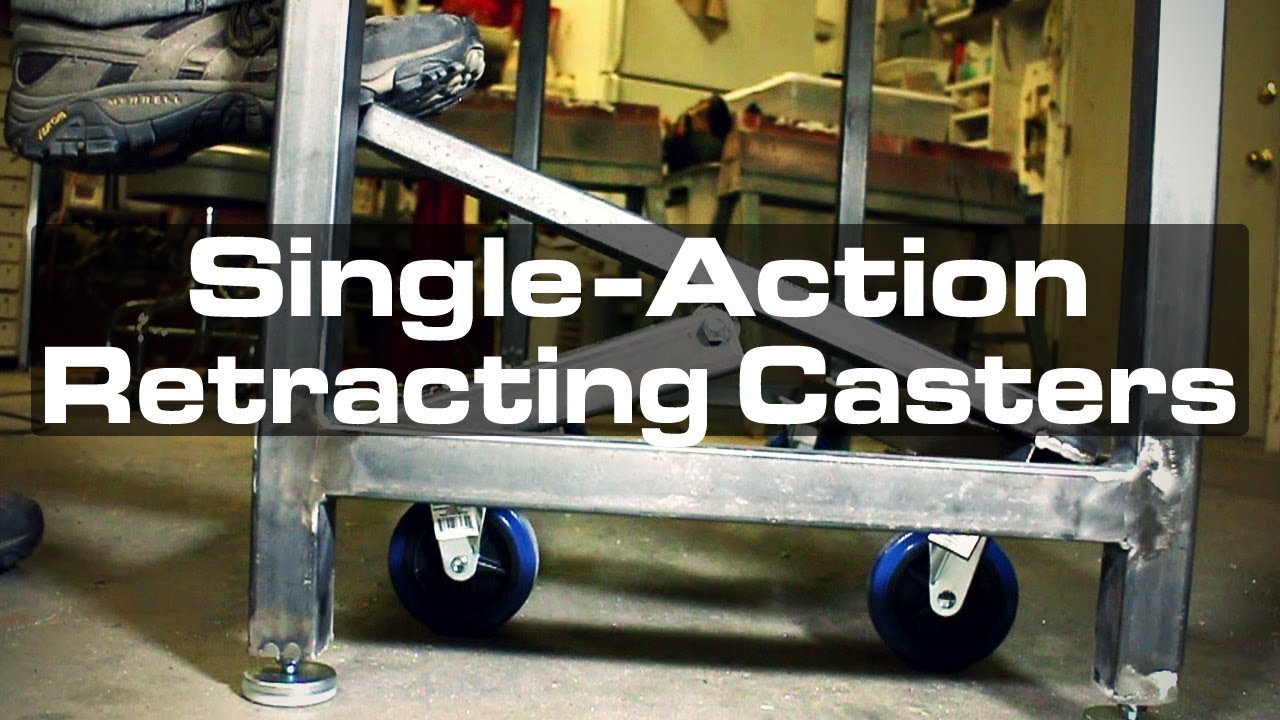In this landscape-oriented photograph, about 1.5 times wider than it is tall, we see a cluttered workspace that could be a workshop or garage. The foreground features a metal cart made of steel or aluminum, structured as a rectangular base with squared-off legs and crossbars forming an H-shape. An angled bar runs from the bottom left to the bottom right, where a man's brown shoe rests. Attached to the cart are two vibrant blue wheels, which are slightly off the ground. In the background, a variety of tools and junk are scattered around, including an old-fashioned refrigerator and a small bar stool. Superimposed in bold, filled-in white text at the front of the image are the words "single-action retracting casters," possibly indicating a demonstration or instructional context for these specific wheels.